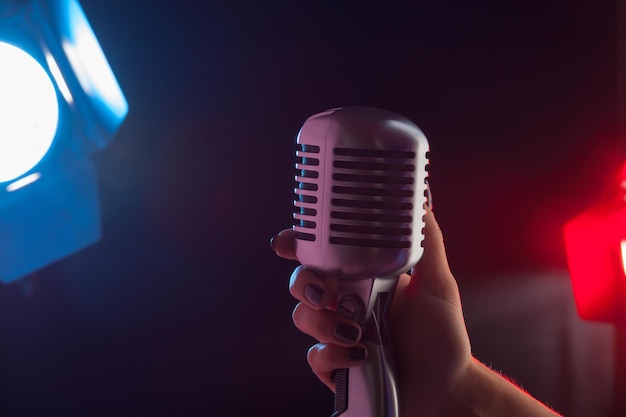The image depicts an up-close photograph of a vintage-style, metallic gray microphone, reminiscent of those from the 1940s, positioned on a stage. The microphone features a silver ball-like top with evenly spaced horizontal lines running from top to bottom. It is mounted on a stand that extends downward, out of the frame. A hand, likely a woman's, is grasping the microphone at its base, showcasing black nail polish against the metallic surface. Two distinct floodlights illuminate the scene: a blue floodlight from the left casts a cool hue on the microphone and the woman's fingers, highlighting the hair on her arm, while a red floodlight from the right bathes the right side of the setting in warm, red tones. The background is dark, enhancing the dramatic effect created by the contrasting red and blue lights, reminiscent of a concert stage.